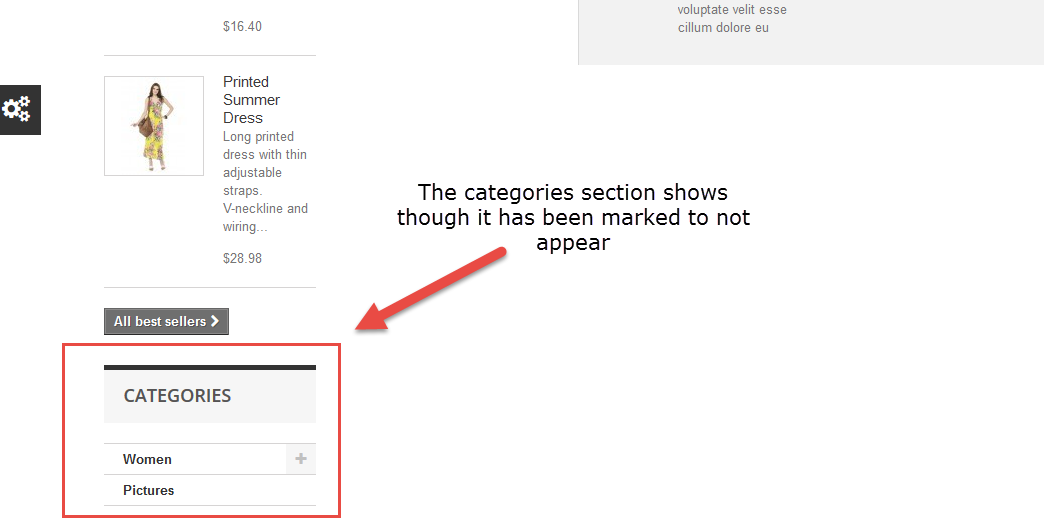The image is a screenshot of a website displaying a product page. At the top of the page, on a gray background with light black font, there is a title in Latin: "Voluptate Velites Cilium Dolore EU." To the left of this title, there is a listed price of $16.40.

Below this section, there is a prominently featured picture of a woman wearing a yellow, printed summer dress. The dress is described as a "long printed dress with thin adjustable straps, V-neck line, and wiring." The woman is holding a bag and has her left hand placed on her waistline. The price of this dress is listed as $28.98 USD.

To the left of the image, there are several gear icons, suggesting options to manipulate the website's settings. To the right of the image and the dress description, a category section is mentioned, but it has been marked to not appear, indicated by a diagonal red arrow pointing downwards.

Further left, there is a navigational section highlighted in a red rectangle, listing options such as "All Bestsellers," "Categories," "Women," and "Pictures."